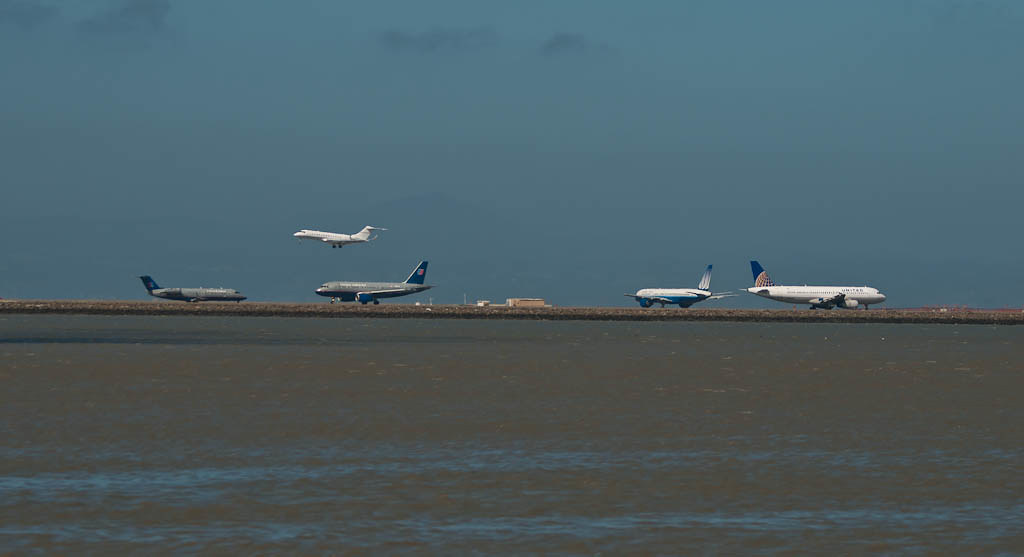This image depicts a bustling airport scene under a hazy, cloudy, and slightly foggy sky with a dark teal hue. The foreground features a murky brownish-blue body of water, while the runway stretches across the middle ground, adorned with several airplanes. On the left side, a white plane is high in the air, appearing to be landing. Below it, two gray planes are situated on separate runways, facing different directions but fairly close to each other. Moving rightwards, another gray plane is seen, followed by two more white planes on the runways that seem to be preparing for takeoff, positioned opposite each other. A United airplane is easily identifiable among them. The far background reveals an airport building, possibly the traffic control tower. The overall atmosphere suggests an overcast, middle-of-the-day setting, giving the airport a busy yet organized appearance.